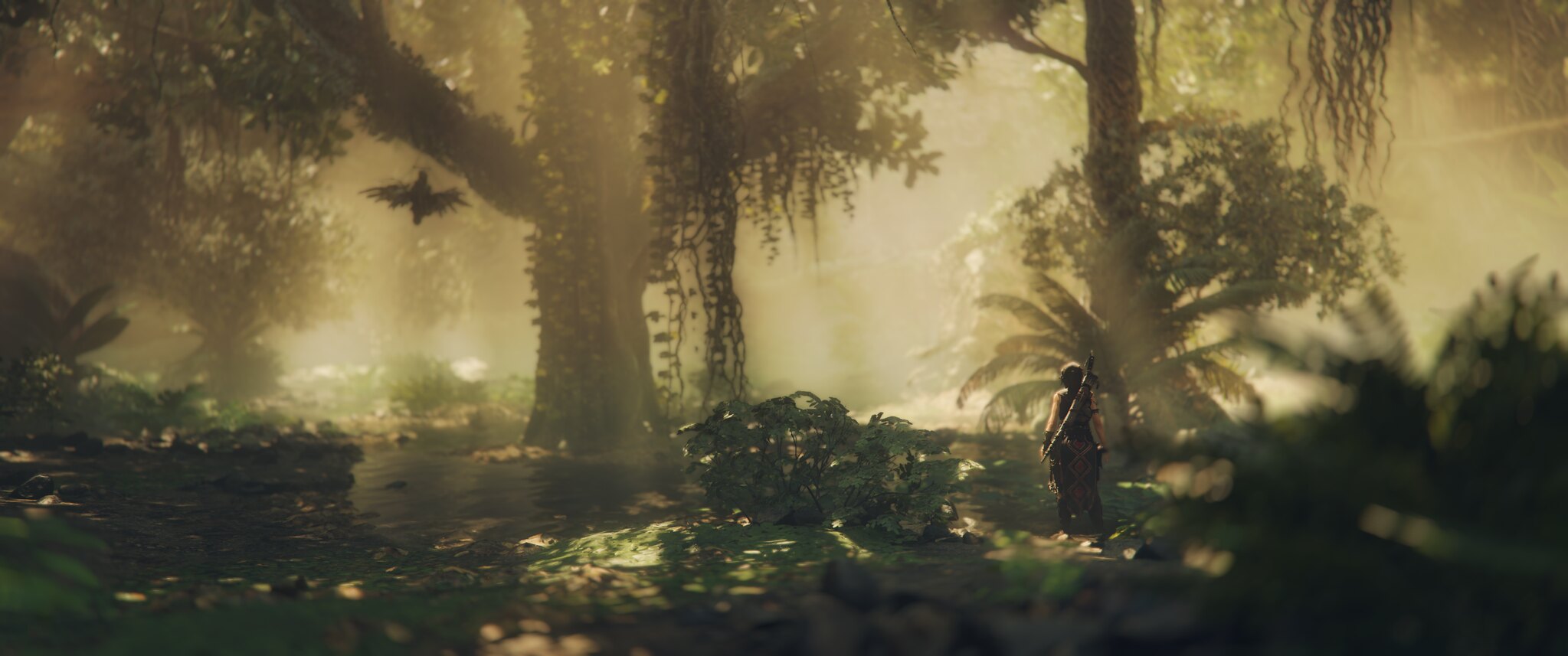This striking drawing depicts a dense rainforest or jungle environment, rendered in a stylized, photorealistic manner with an intriguing palette of predominantly brown and olive green shades. At the center of the scene, a large tree with a massive trunk commands attention, flanked by another substantial tree to its right. Both trees are draped with vines and possibly Spanish moss, contributing to the dense forestation. An assortment of large ferns or palms can be seen, adding to the lushness of the forest floor, which is covered in various undergrowth including leaves and bushes.

A subtle light suggests an opening in the canopy, allowing rays of sunlight to peek through, casting soft shadows on the ground. Off to the left of the central tree, a bird with a large wingspan, possibly a vulture, is perched, adding a dynamic element to the composition. On the right side, in the distance, there is the faint silhouette of a person standing, appearing to observe the forest. Closer inspection reveals this figure might be equipped with a sword on their back, increasing the narrative intrigue of the scene.